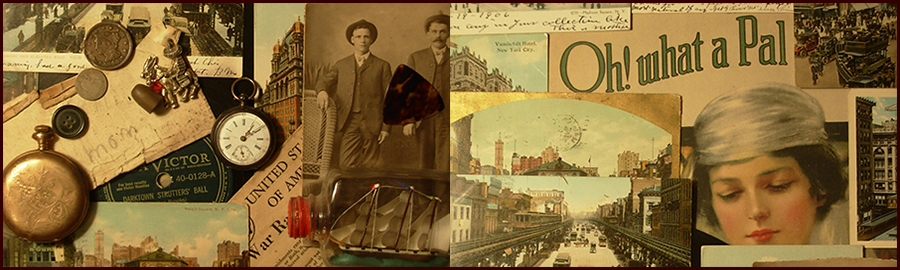This long, rectangular collage holds an assortment of vintage images and objects, predominantly from the early-to-mid 20th century. Dominating the left side, there are a couple of bronze pocket watches positioned on a folded piece of paper bearing the word "mom." Surrounding them are old tins, postcards, buttons, and perhaps an antique penny, evoking a nostalgic aura. Central to the collage, black-and-white photographs depict people dressed in antiquated suits, alongside other historical snapshots. A notable addition is a ship encased in a glass bottle with a red lead, accompanied by a small note reading "oh what a pal" in green, lying adjacent to images of a bandaged woman and a cityscape featuring a girl with a fashionable hat. The various elements, including coins, a guitar pick, and buttons, suggest a curated reflection of a bygone era, encapsulating fragments of someone's life and memories.